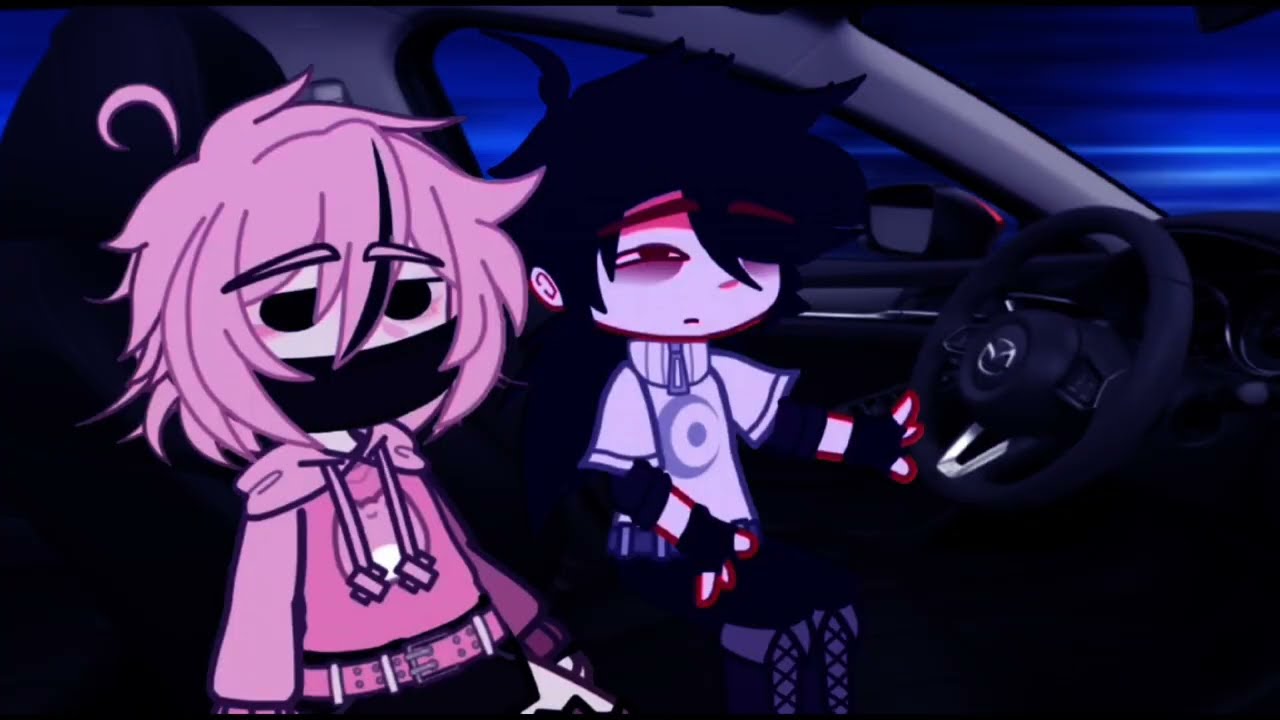In this detailed and descriptive caption, emphasis is placed on the shared and repeated elements from the three sources:

The image depicts two anime-style cartoon characters seated in the front of a car, which seems to be either a Lexus or Mazda, indicated by a partial view of a logo on the black steering wheel. The scene is set at night, with a dark blue sky visible through the car windows. 

In the driver's seat, a boy with pale skin and black hair appears somber, his eyes mostly closed. He is dressed in a white and blue short-sleeved shirt featuring a circular logo with a quarter moon inside, black pants, and purple boots. His left hand rests on the steering wheel.

Next to him in the passenger's seat, a girl with messy chin-length pink hair and shades of pink attire is visible. She wears a pink hoodie adorned with an animal graphic, a pink belt, and black bottoms. Her face is partially covered by a black mask, and her large black eyes stare ahead.

The car's interior includes black seats and contrasting white interior walls, contributing to the dimly lit, mysterious atmosphere inside the vehicle.